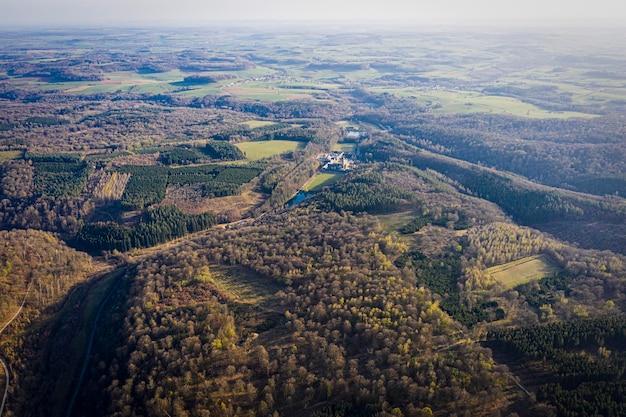This aerial photograph captures a sprawling, forested landscape characterized by rolling hills and open green fields. The dense forest dominates the scene, with various shades of green showcasing treetops, interspersed with patches of slightly browning vegetation, hinting at early fall. The top half of the image reveals hilly terrain, transitioning to flatter land as it descends. A thin road cuts through the forested lower left corner, winding its way towards the center. Here, a small cluster of buildings, discernible by their grayish-white hue, is positioned near a small body of water. Additional roads can be seen extending left to right and further through the foliage in the bottom third of the image, adding to the complexity and charm of this richly textured landscape.